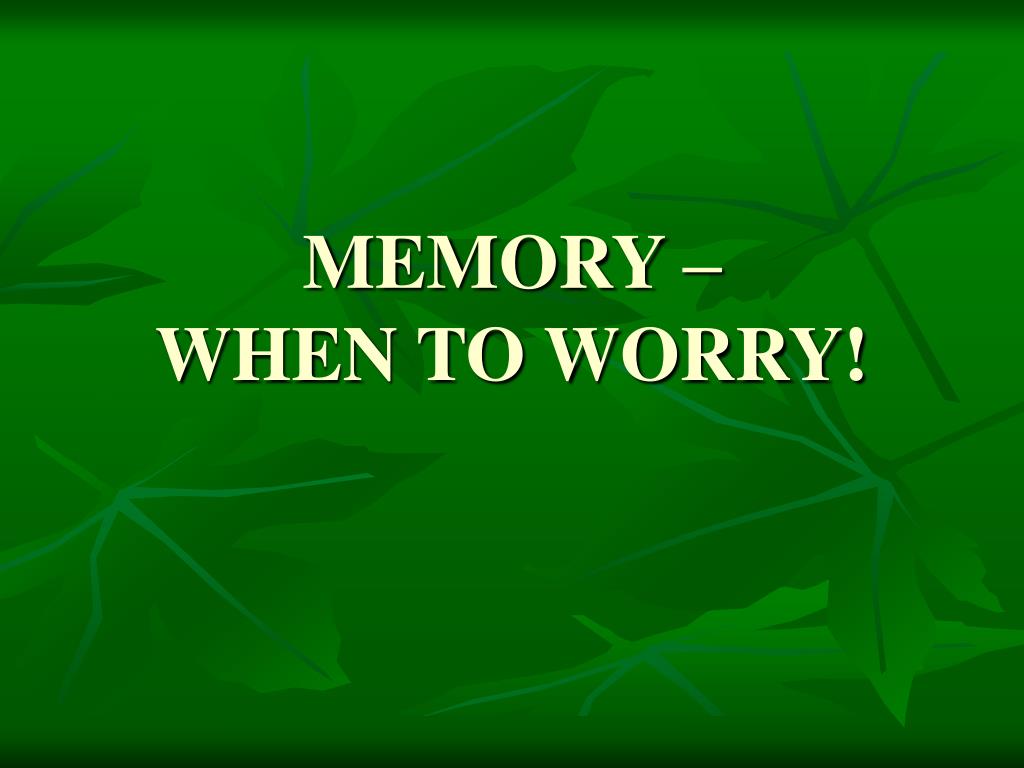The image is a digital artwork featuring a predominantly green background with an overlay of six green leaves, each having a lighter green shade for the veins. In the center of the image, in bold all-capital letters, are the words "MEMORY - WHEN TO WORRY!" in white font, outlined by a black shadow or border, creating a striking contrast against the green backdrop. The graphic design seems intended for a PowerPoint presentation, possibly discussing aspects of memory and when to be concerned about memory issues. The leaves are arranged with some overlapping at the bottom right corner, adding depth to the composition.